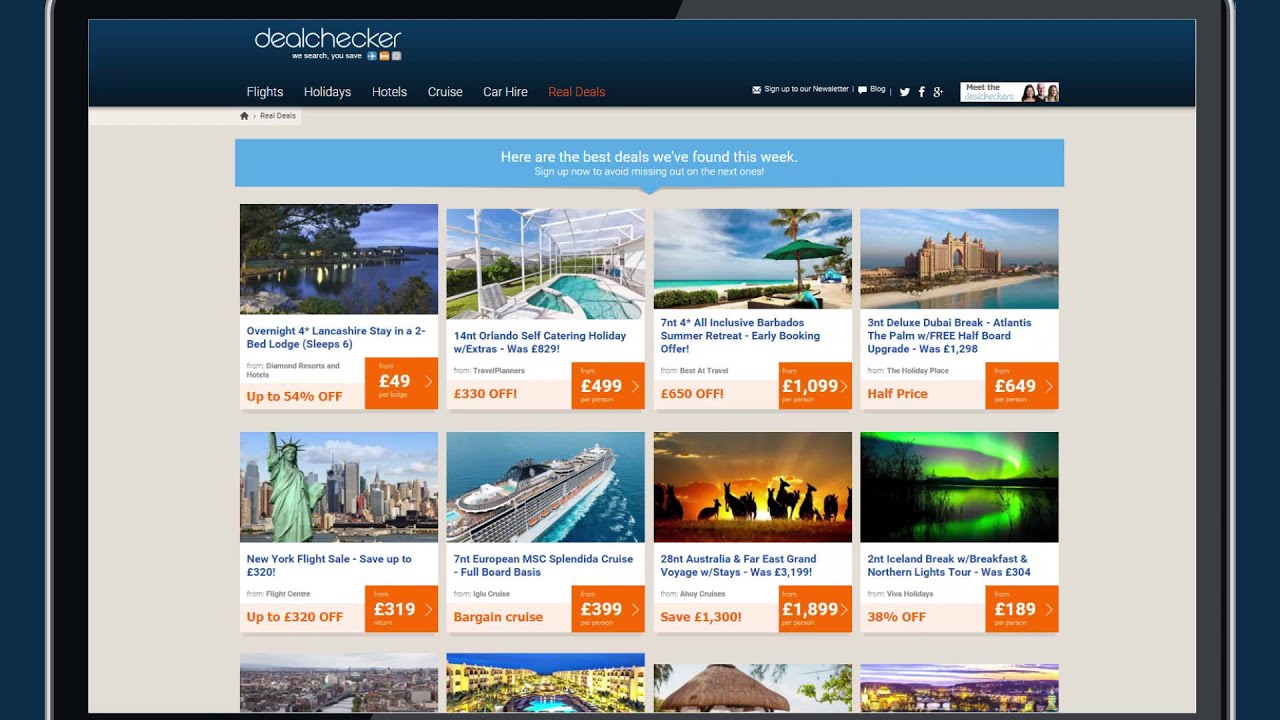This image is a detailed zoom-in of an advertisement from the "Deal Checker" website, displayed on what appears to be a laptop or tablet screen. The top portion of the image features a dark blue banner. Dominating the banner is the name "Deal Checker" in prominent white text. Directly beneath this name, in smaller white letters, the categories “Flights,” “Holidays,” “Hotels,” “Cruise,” and “Car Hire” are listed, indicating different sections of the website. In contrast, the phrase “Real Deals” is presented in striking red text. 

On the right side of the banner, smaller white text reads, “Sign up to our newsletter, blog,” accompanied by icons for social media platforms Twitter, Facebook, and Google+. Below this, there’s a small advertisement with the tagline, "Meet the Deal Checkers," showcasing images of several individuals.

The main portion of the advertisement focuses on impressive lodging deals. For example, on the top left, there’s an offer for an "Overnight Lancashire stay in a two-bed lodge, sleeps six for £49," boasting a savings of up to 44%. To the right, another deal highlights a "14-night Orlando self-catering holiday with extras," reduced from £829 to £499, offering a substantial saving of £330.